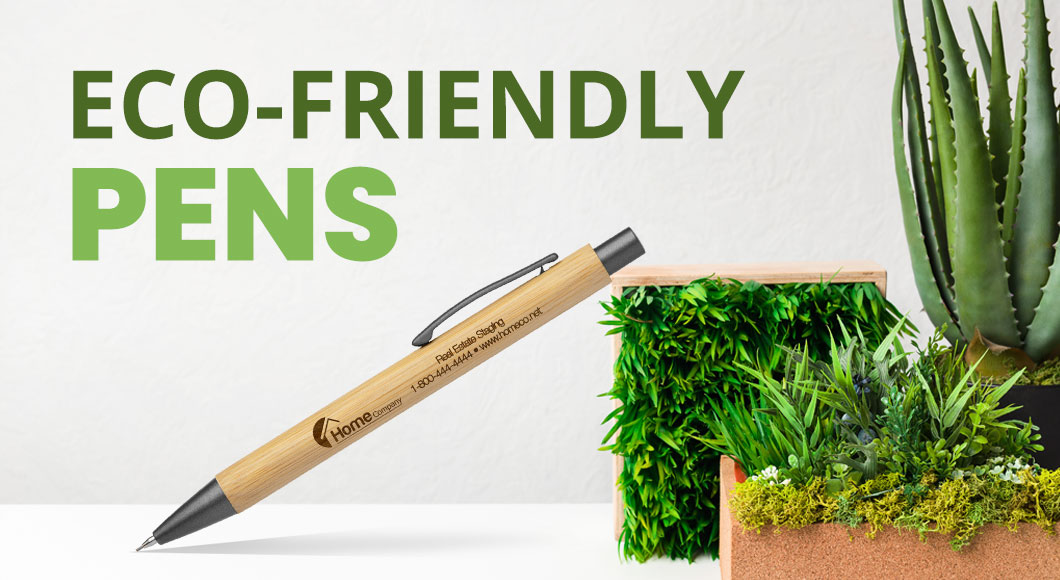The image is a detailed product photograph set against a white or light blue background. Central to the composition is a bamboo pen positioned diagonally, with its gray tip pointing towards the bottom left corner and the gray plunger end located near the center. The pen, bearing brown text, features the logo "Home Company Real Estate Staging" along with a contact number and web address. Propped on a square wooden planter filled with green plants, the pen casts a shadow that adds depth to the scene. To the right, another similar square wooden box displays more plants, including an aloe plant. At the top left corner of the image, the words "ECO-FRIENDLY" in all-capital dark green letters are prominently featured, with "PENS" below it in a larger, lighter green font. The photograph is distinctly focused on realism, showcasing the eco-friendly nature of the pen amidst a natural setting of plants.